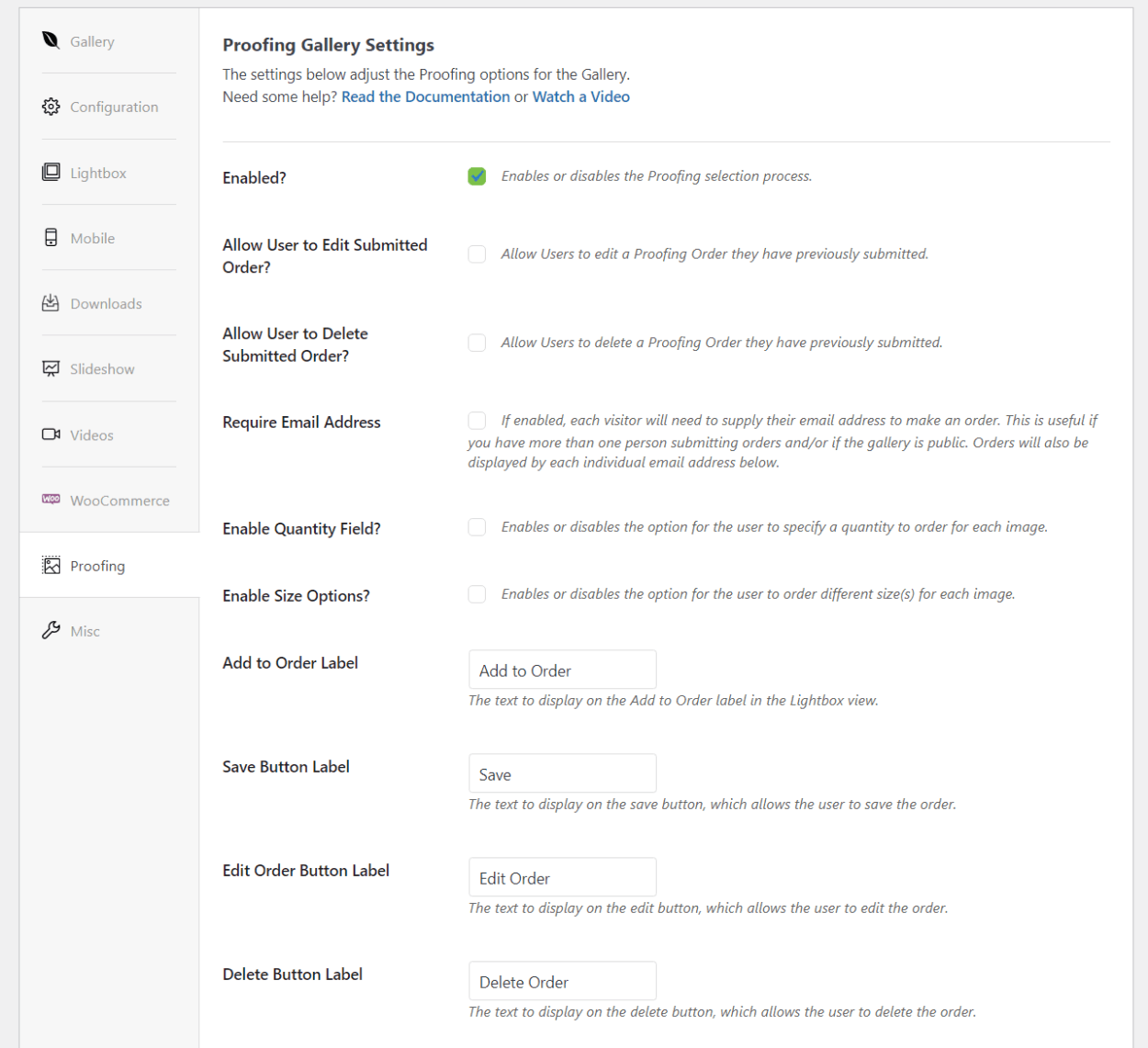This is a detailed screenshot of a computer interface displaying a comprehensive settings menu for a proofing gallery within a software application. On the left-hand side, there is a vertical menu with various options, each accompanied by a small icon. The options listed are: Gallery, Configuration, Lightbox, Mobile, Download, Slideshow, Videos, WooCommerce, Proofing, and Miscellaneous. The active selection is 'Proofing,' and its corresponding settings are displayed on the main part of the screen.

At the top of the main section, it reads 'Proofing Gallery Settings,' followed by the subtext: "The settings below adjust the proofing options for the gallery. Need some help? Read the documentation or watch a video." The phrases "read the documentation" and "watch a video" are highlighted in blue while the rest of the text remains black.

Beneath this introductory text, there are various configuration options starting with an 'Enabled' option, indicated by a green checkmark, which states that it "Enables or disables the proofing selection process." The subsequent settings include:

- Allow user to edit submitted order
- Allow user to delete submitted order
- Require email address
- Enable quantity field
- Enable size options
- Add order label
- Save button label
- Edit order button label
- Delete button label

Each of these settings provides detailed information about its function. The overall color scheme of the interface is primarily black and white, with the settings menu on the left presented in a light gray box. The user has clicked on the 'Proofing' option, which is why related settings are prominently displayed in the central portion of the screen.